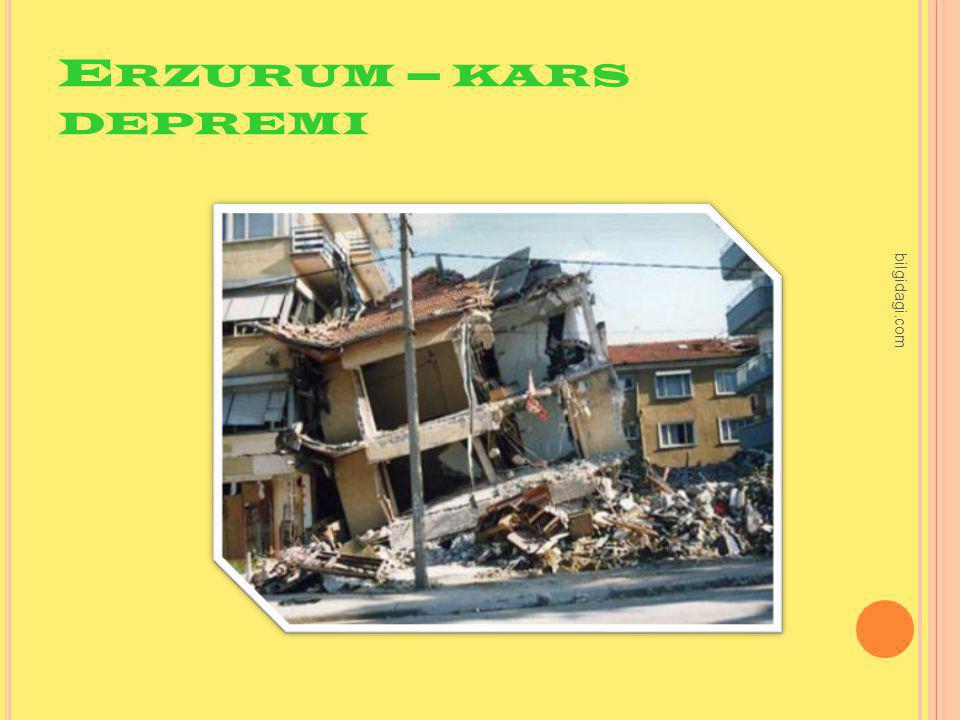A photograph centrally framed within a white border and a larger yellow border showcases the aftermath of a catastrophic event. The yellow border features green text at the top, reading "ERZURUM-KARS F-DEPREMI," indicating the likely location and nature of the disaster. On the right edge, a thin peach-colored line runs vertically, accompanied by black text that reads "BILGIDAGI.com." Also on the yellow border, an orange circle is positioned near the bottom right corner.

The central photograph depicts a severely damaged building, which is notably collapsed and missing much of its front facade. The left side of the building remains somewhat intact with a tiled roof and appears to be a two-story structure. In contrast, the right side has completely collapsed, exposing concrete, rebar, and debris scattered across the street below. The destruction has even caused the building to lean into an adjacent apartment building. Surrounding the scene are other buildings and an electricity line, set against a blue sky, adding to the abandoned and chaotic atmosphere of the image. The overall composition, with its detailed borders and vivid depiction of the aftermath, suggests an informational or news-reporting style, possibly documenting the damage from a natural disaster.